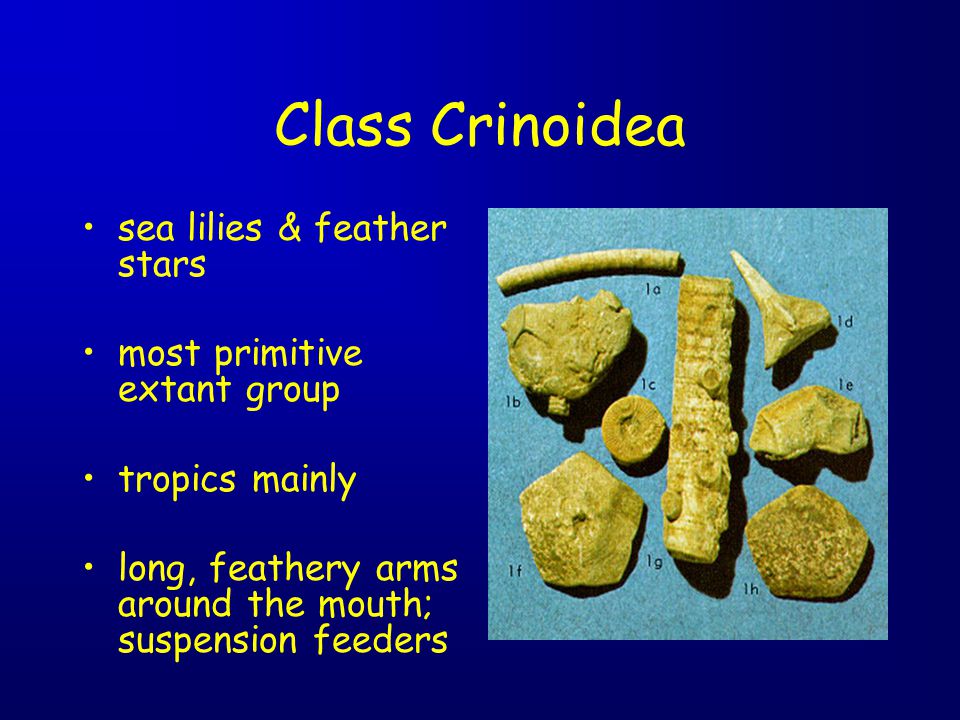The image resembles an educational slide, likely part of a PowerPoint presentation, set against a dark blue background that fades lighter towards the top. Dominating the slide is a mix of text and a photograph. At the top center, in bold yellow text, the title reads "Class Crinoidea" with red dotted lines surrounding the word. 

To the left, there are four bullet points in smaller yellow text, listing:
1. Sea lilies and feather stars
2. Most primitive extant group
3. Tropics mainly
4. Long, feathery arms around the mouth; suspension feeders

The right side features a photograph on a light blue background, showcasing several fossilized bones and teeth, labeled 1A through 1H. The central object within the photograph appears to be a long cylindrical item surrounded by various pieces of rock, potentially archeological tools or fossils.